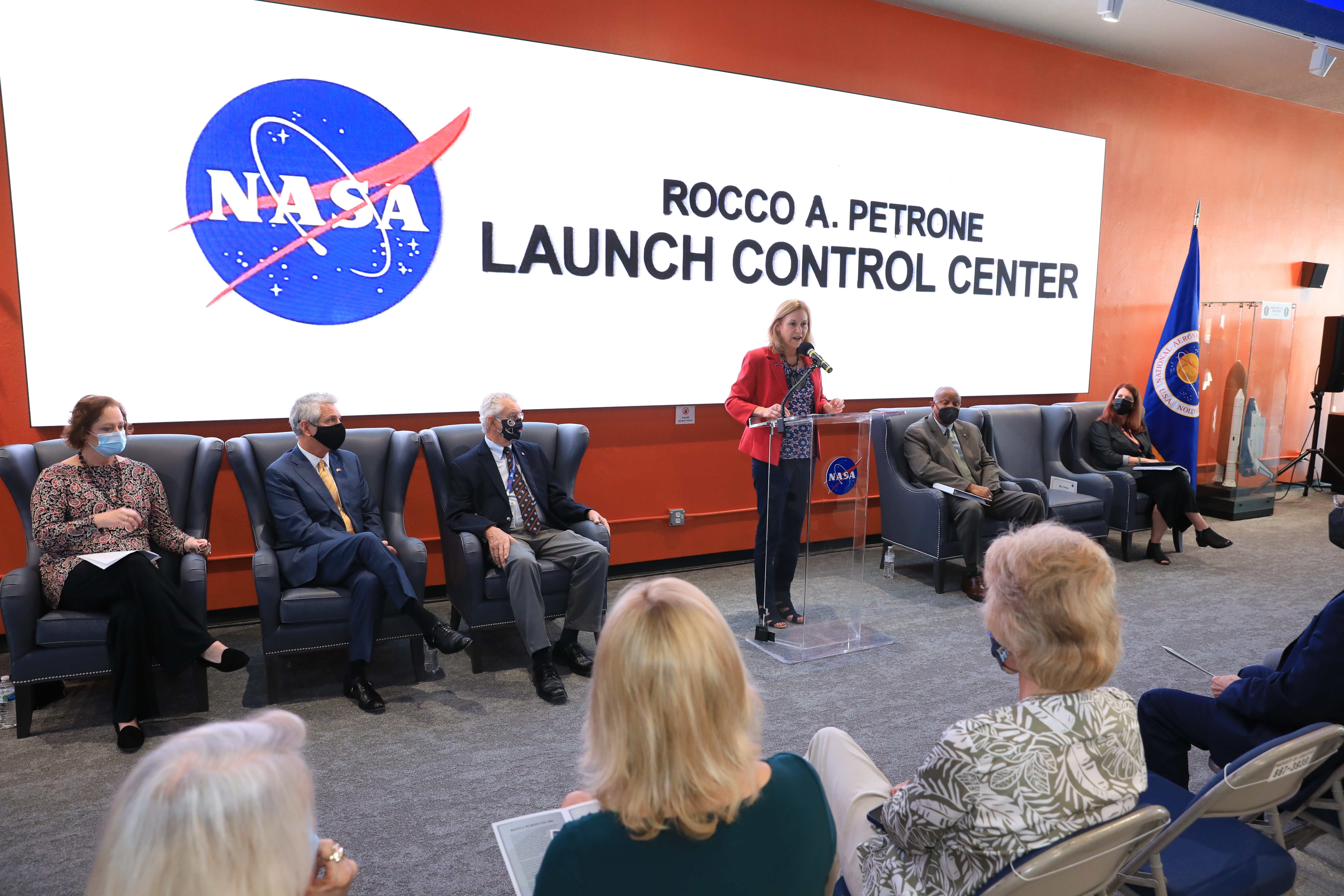In the photograph, a blonde woman with shoulder-length hair is giving a presentation at a clear podium emblazoned with the NASA logo, a blue circle with white letters and a red chevron. She is dressed in black pants, a blue shirt, and a red jacket, and is speaking into a microphone. Behind her, a large screen displays the text "Rocco A. Patron Launch Control Center" in black letters on a white background, flanked by the NASA logo to the left. The event seems to be held during the height of the COVID pandemic, as all attendees are wearing masks. In the audience, dignitaries are seated on comfortable couches on either side, while others, possibly older women, sit attentively on folding chairs in front of her. The surroundings feature a red-painted wall, adding vibrancy to the scene, and a NASA flag displayed to the right of the podium. The speaker appears to be addressing the status of a launch, given the context of the Launch Control Center.